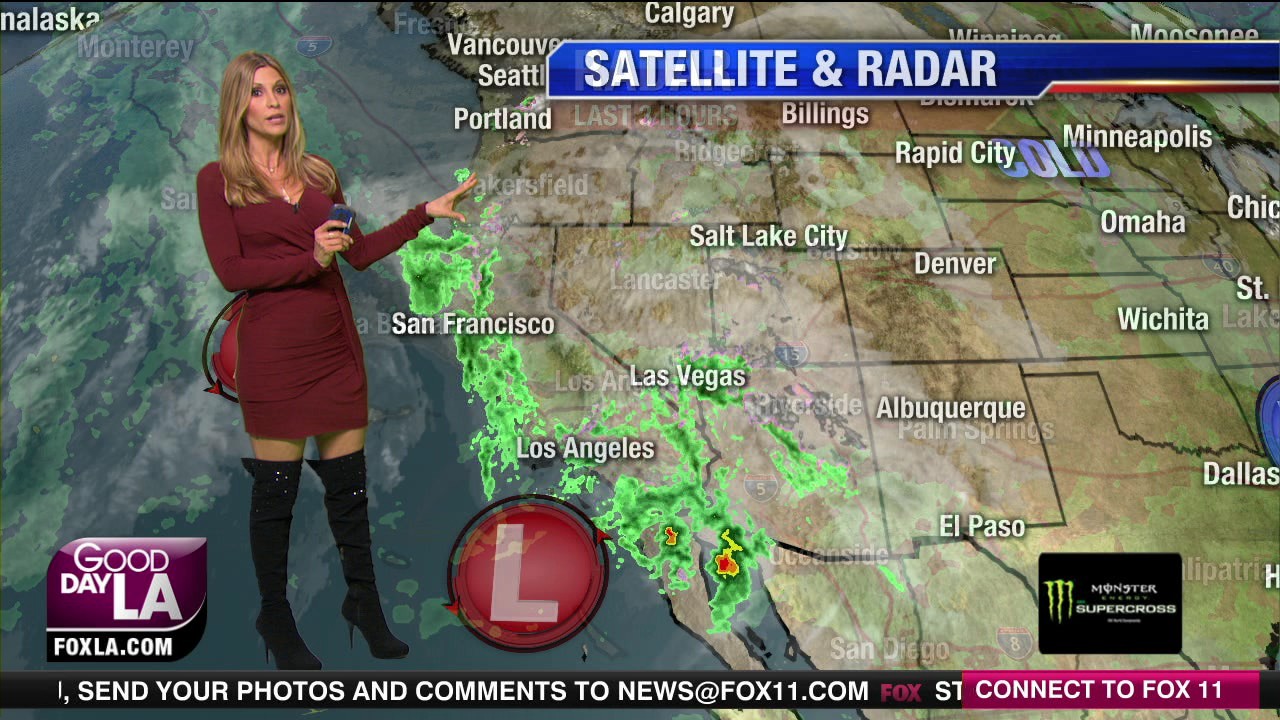The image depicts a female weather forecaster delivering the weather on TV. She is a white woman with long, dirty blonde hair that extends past her shoulders and is dressed in a maroon or red dress that falls just above her knees, paired with tall, black high-heeled boots. She is positioned to the left of the image, facing forward while slightly turning to the right, with her left hand pointing to a weather map and her right hand holding a black object near her body. The weather map covers the United States, emphasizing the western part, and prominently features a green precipitation area near Northern California, including cities like San Francisco and Portland. The map extends from Calgary at the top to Dallas on the right edge and shows a circle with a red center and white 'L' below Los Angeles. At the top of the map, in white lettering on a blue background, it reads "Satellite and Radar." The bottom left of the image displays the text, "Good Day LA, FoxLA.com," while a ticker tape at the bottom advises viewers to send their photos and comments to news@fox11.com and to connect with Fox11.